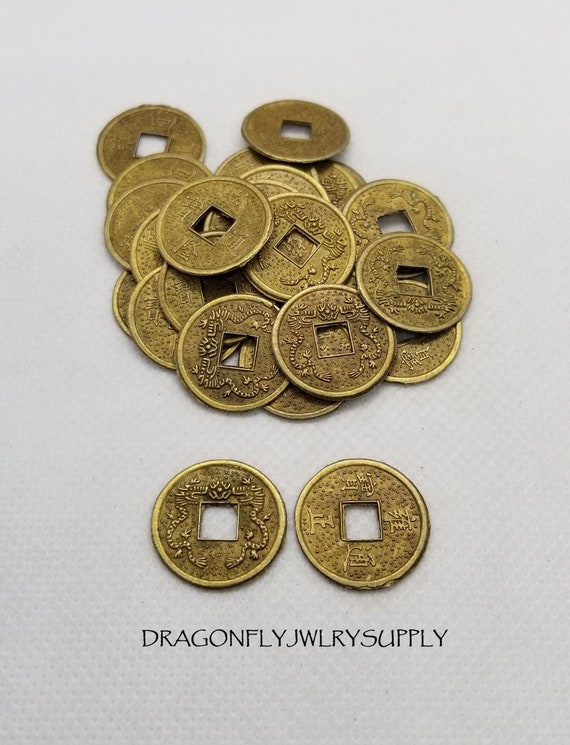The image features a collection of round, gold-colored disks that resemble coins, each with a square hole cut in the center. The coins are intricately designed with Chinese-style elements: one side displays two dragons on either side of the square holes, while the reverse side features four Chinese characters positioned around the square. The coins are arranged with some laying flat and others in a small pile towards the top of the image. The background is a textured gray surface, similar to a paper towel but not actually one. Positioned along the bottom of the image, in black font, is the name "Dragonfly Jewelry Supply," with "Jewelry" abbreviated as "Jwlry." This branding indicates that the coins are likely part of a jewelry supply collection rather than actual currency.